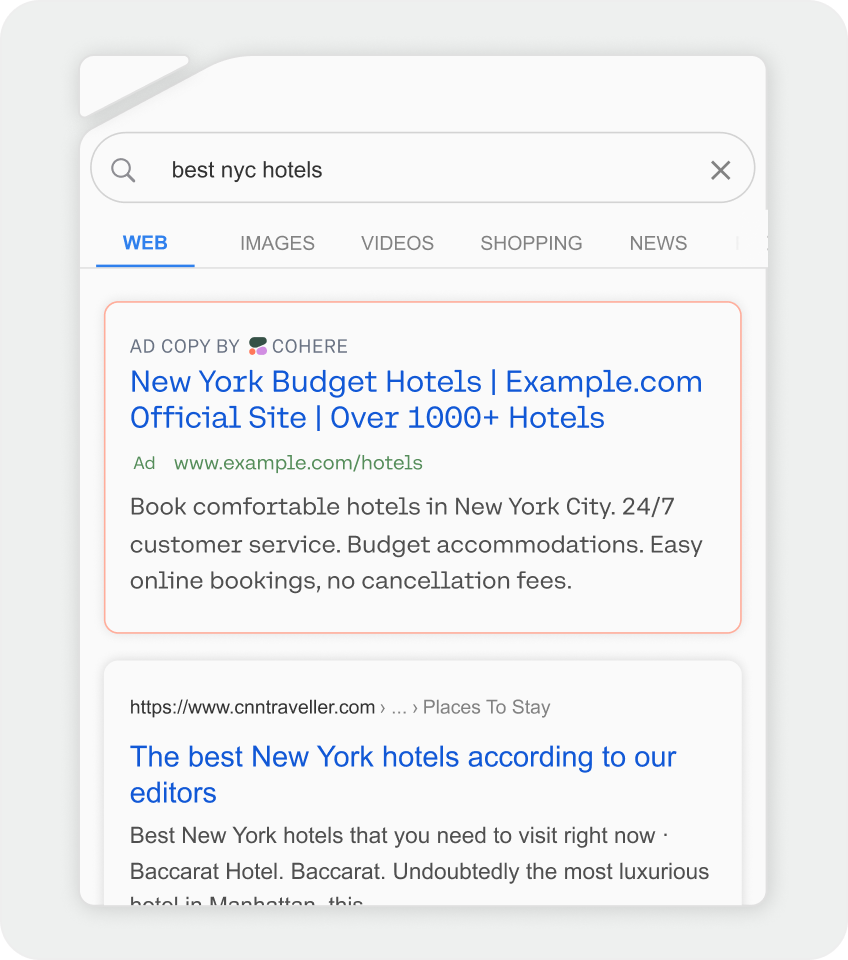This image displays a search results page from a mobile phone, set against a light gray background with a faint shadow for depth. The main content is presented on a white, rounded-cornered rectangle, suggesting a sleek and modern user interface. 

In the top left corner, a small triangular segment is cut out, revealing the light gray background behind it, which forms an angular detail at the top left of the main page. 

At the very top, there's a white search bar bordered with a thin light gray outline. Within the search bar, a magnifying glass icon is positioned on the left, an 'X' is on the right, and the phrase "Best NYC Hotels" is typed in black text. Just below the search bar are navigation tabs: "Web" highlighted in blue and underlined, followed by "Images," "Videos," "Shopping," and "News" in gray.

A subtle gray line runs horizontally beneath these tabs, aligning with the blue underline of the "Web" section.

The search results are presented in two distinct sections, each with a white background, rounded corners, and thin borders. The top section is outlined with a very thin orange line. In the top left corner of this section, light gray text reads "Ad Copy by Cohere," accompanied by a small logo consisting of three colorful shapes. Below this, in blue text, it reads "New York Budget Hotels example.com official site over 1,000+ hotels," followed by a green text link "Ad www.example.com/hotels."

Further details describe: "Book comfortable hotels in New York City, 24/7 customer service, budget accommodations, easy online bookings, no cancellation fees," in gray text, succinctly highlighting the service features.